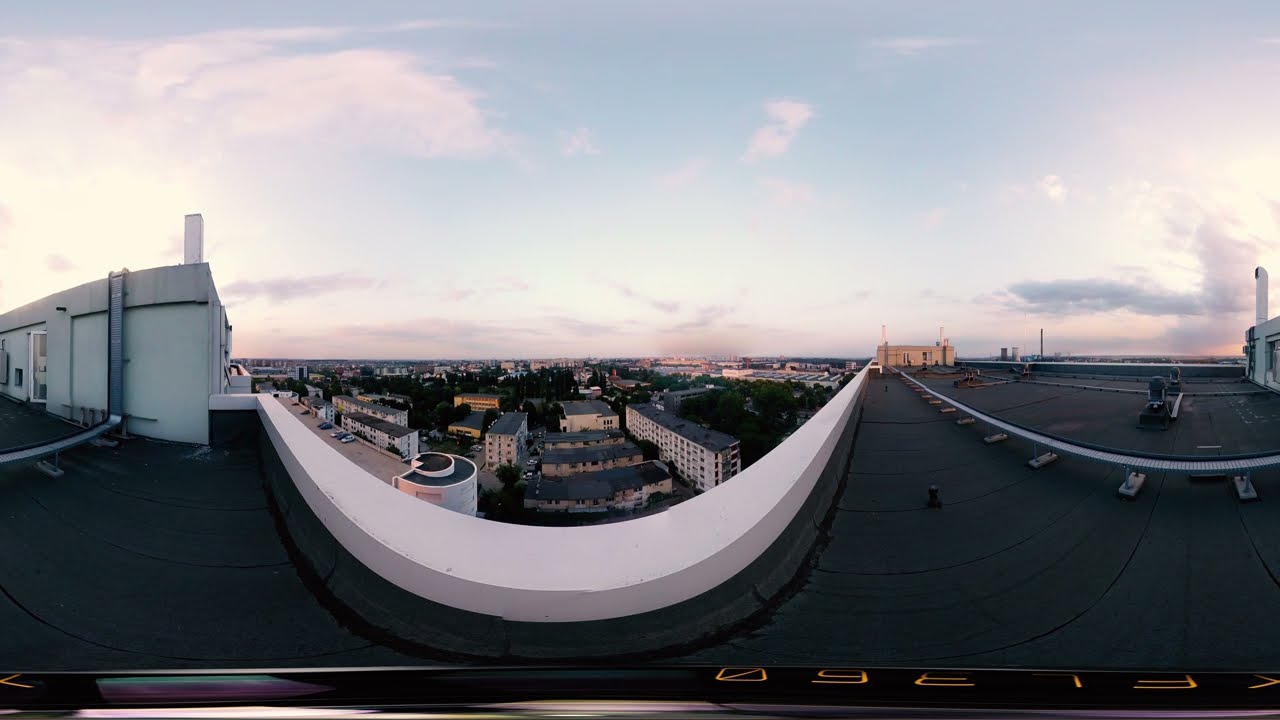This detailed photographic image captures an expansive outdoor cityscape through a fisheye lens, creating a slight curved distortion. The picture is taken from the vantage point of a rooftop of a multi-storied building, revealing a broad view of various types of buildings below, including residential, industrial, and commercial structures. The rooftop, covered in black tar with a white border to prevent falls, features a glass door on one side. To the left, there is a square-shaped structure with a ladder leading to a doorway. The scene includes a street on the left side with cars parked, and buildings with grey roofs. Notably, there is a tall granite building in the far background to the right, and closer by, several industrial structures including a smokestack and white and grey chimneys. The sky occupies the top half of the image, transitioning from light blue at the top to a whiter gray near the horizon, dotted with varying shades of clouds from white to dark gray. The time of day appears to be around sunset or sunrise, as indicated by the lighting and the partly obscured sun seen against some clouds. Additionally, the letters "K-E-I-6-N" are faintly visible in the bottom right corner.